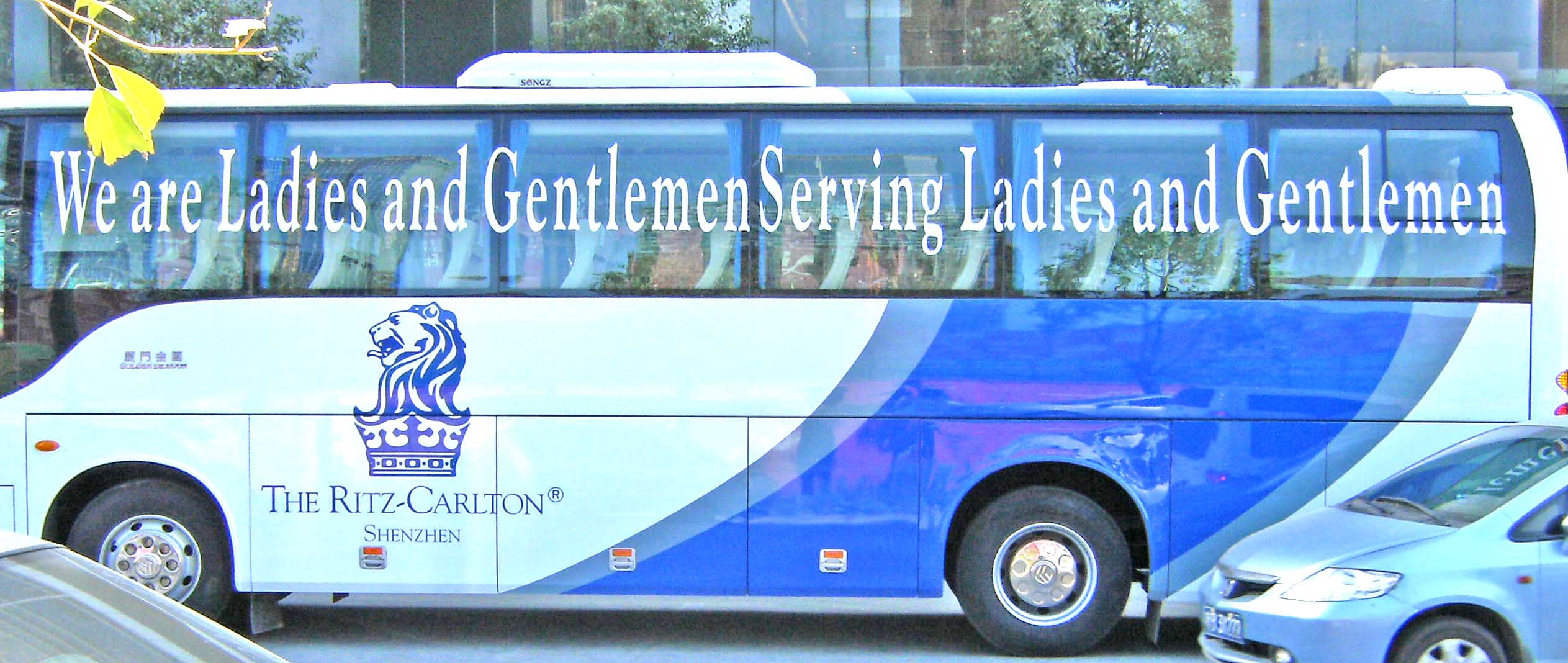The image depicts a large white bus with a blue stripe toward its rear, captured outdoors during the daytime. Prominently displayed on the side of the bus is the slogan, "We are ladies and gentlemen serving ladies and gentlemen," attributed to the Ritz Carlton, Shenzhen, suggesting a possible Chinese location. The text appears to be printed on the window, though some elements may have been digitally enhanced. Adjacent to the slogan is an artwork featuring a lion's head with a crown, notable for its blue and purple coloration. The bus occupies most of the frame, with trees towering in the background, their lush green foliage visible above the vehicle. To the right bottom corner of the image is a light blue car, while the windshield of another car is barely visible in the left bottom corner. In the top left corner, a stem with leaves can be seen, further enhancing the outdoor ambiance of the scene.